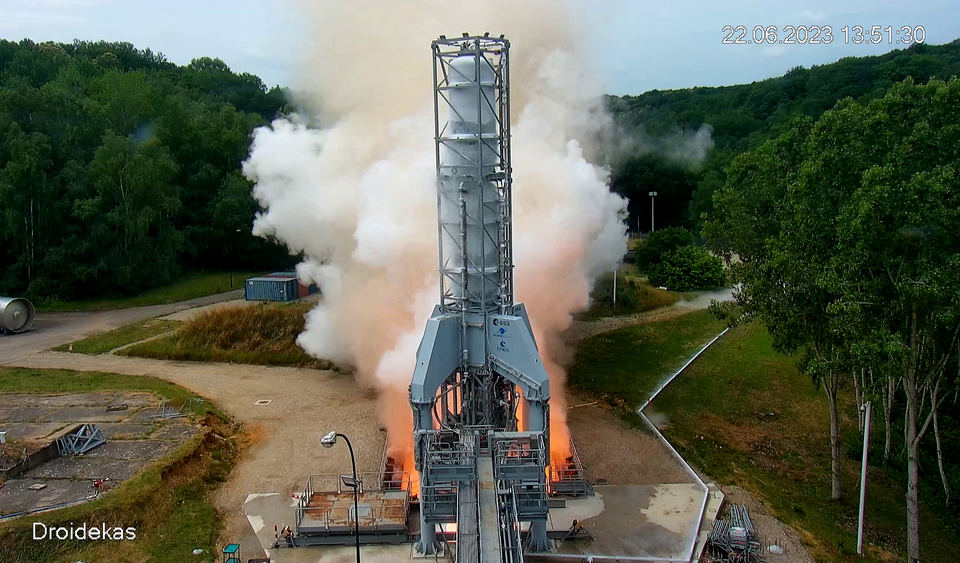In the image, there is a white rocket with a gray and blue base, appearing to be in the early stages of launch, with smoke and steam billowing from its bottom. The scene captures the rocket at the center of what resembles a test facility, featuring a steel catwalk for access. The surroundings include lush greenery, trees, and a dirt roadway under a partly cloudy blue sky. Notably, there is a timestamp watermark at the top right indicating the photo was taken on June 22, 2023, at 13:51:30. At the bottom left, another watermark reads "Droidekas," clearly spelled out as D-R-O-I-D-E-K-A-S.